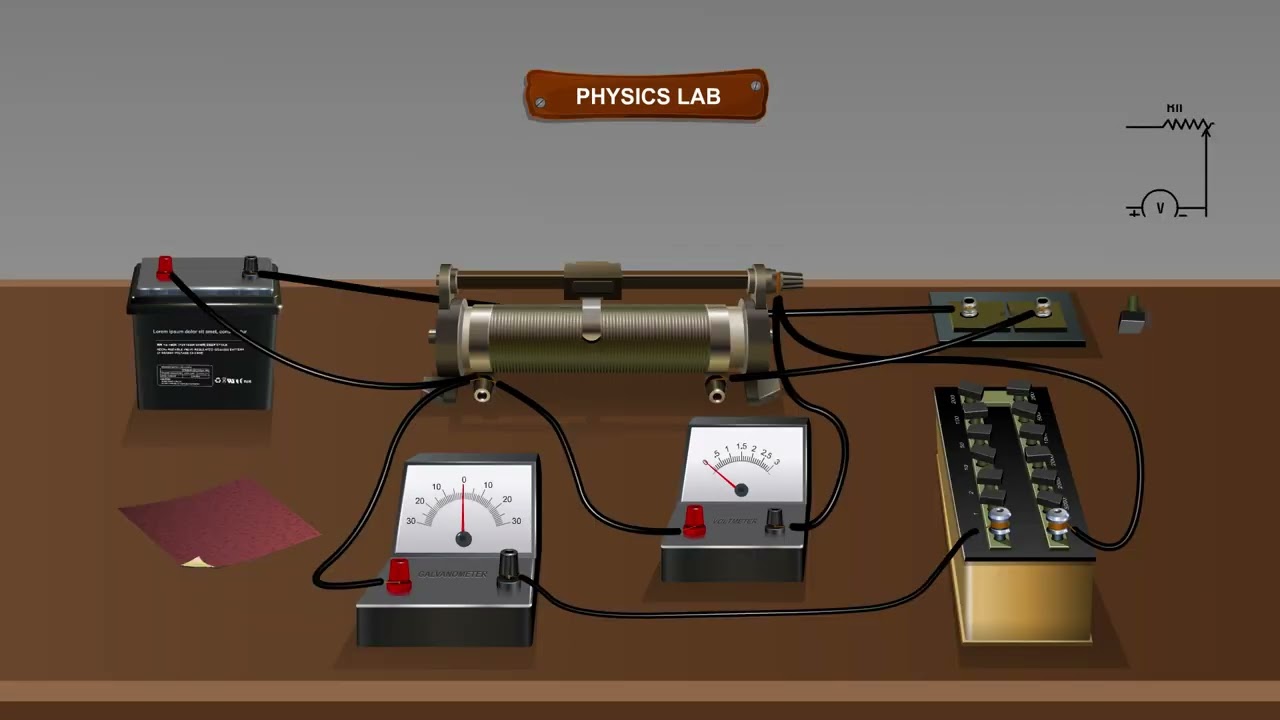This is a detailed digital rendering portraying a vintage physics lab setup. Dominating the background is a gray wall adorned with a russet sign, featuring white text that reads "Physics Lab," possibly resembling a wooden plaque, affixed with two nails. Adjacent to this sign on the right side of the wall is an intricate black electrical circuit diagram.

In the foreground, a brown desk is laden with an array of aged electronic devices. Among the equipment, there is a small black battery with distinct red and black posts, and a green-copper cylindrical machine. Two prominent meters—reminiscent of old-fashioned speedometers—display numerical readouts and are equipped with black and red battery poles. Additionally, there is a black and gold apparatus that appears to be a power outlet. Scattered across the desk are various wires connecting these devices, alongside a conspicuous piece of red paper. The overall scene evokes the ambiance of a mid-20th century physics laboratory, complete with elaborate gadgetry and meticulously detailed circuits.